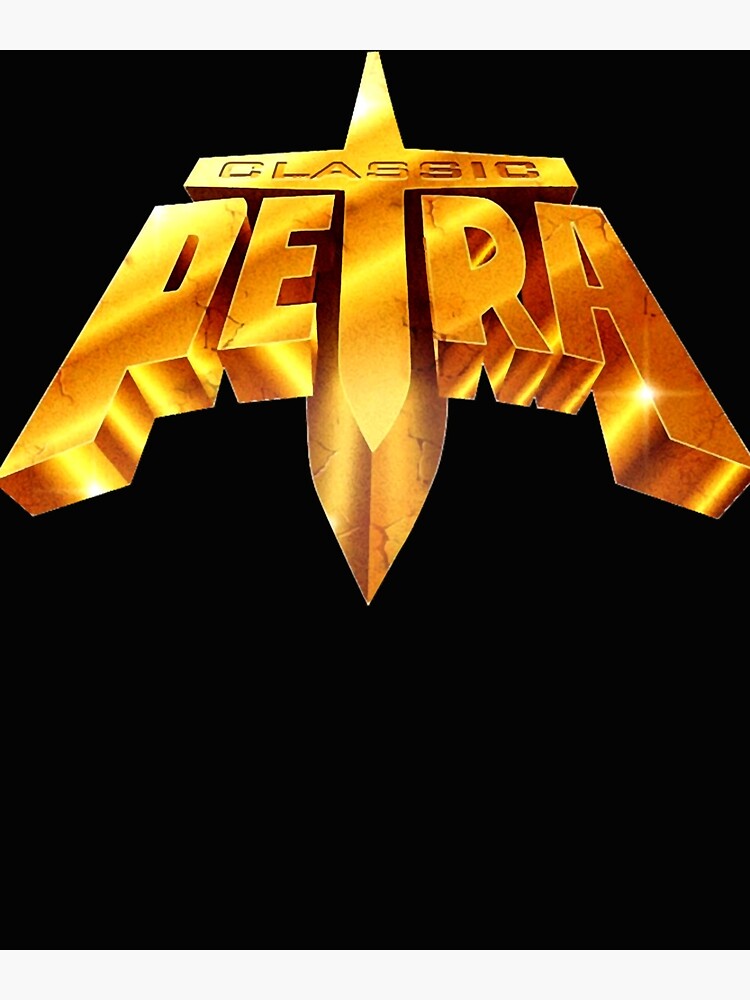The image resembles an album cover with a solid black background. Dominating the top, there's a large, stylized "Petra" symbol that appears to be floating in space. The lettering is bold and gold, glistening in parts as if it were made of shiny gold bricks, with orange shadows accentuating its form. The "T" in "Petra" is uniquely designed to resemble either a cross or a sword, depending on one's perspective, with the word "classic" emblazoned across the crossbar of the sword. The letters of "Petra" are positioned creatively, with "PE" on the left of the sword and "TRA" on the right, extending down to match the lengths of the letters. There are no other elements, such as people or animals, in the image, and several letters feature crack marks, adding to the intricate design. The overall style and rendering strongly evoke the aesthetics of 70s and 80s album art, making it plausible that this is indeed a cover for the band Petra.